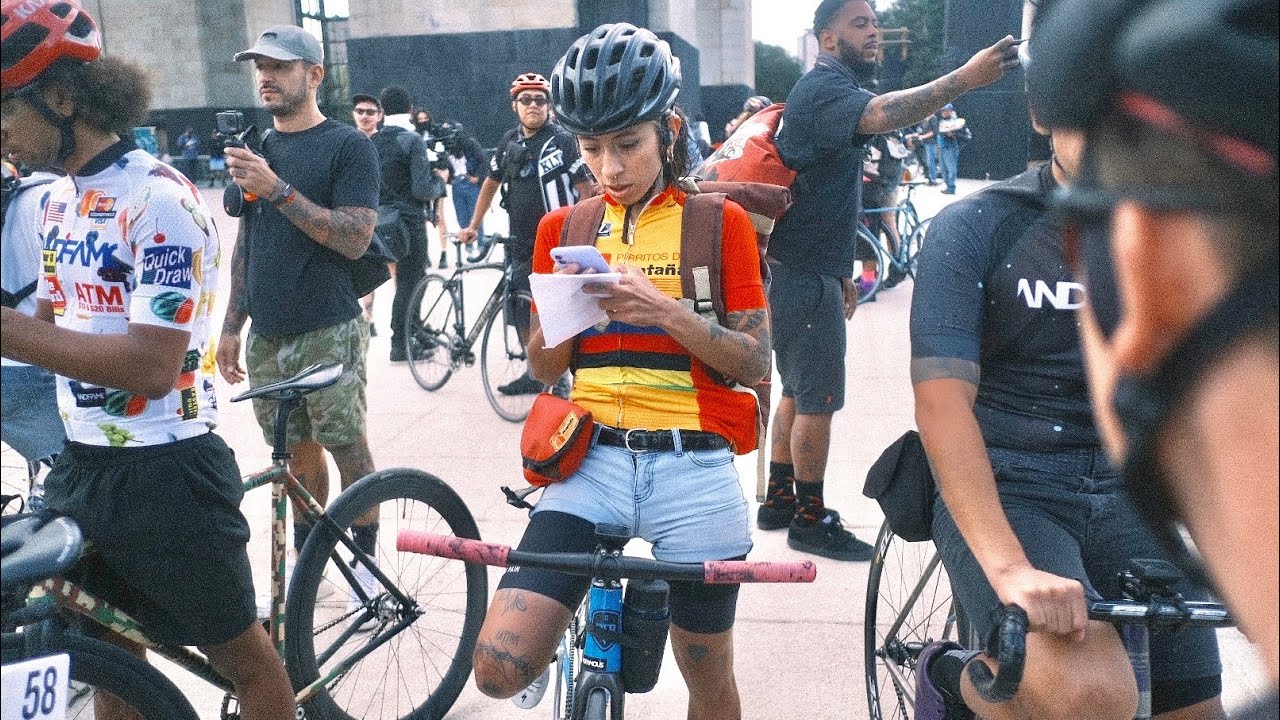In a grainy, deliberately stylized photograph, we see a bustling scene either before or after a marathon bike race, likely taking place on an overcast summer day. Central to the image is a young woman in her late 20s or early 30s, standing idly with her bike. She wears a bright yellow cyclist’s top with orange accents, blue jean shorts over cycle shorts, a black belt, and a black helmet. She is engrossed in her phone, holding a small piece of paper in her hand, possibly looking up race information. Her bike, distinguishable by its red handles, is secured between her legs. 

Surrounding her are other cyclists, all wearing helmets and sporting a mix of shorts and colorful, sporty t-shirts. There is a notable competitor donning the number 58 on his bike's front tire. To her left, a cyclist in a white shirt adjusts his helmet, and to the right, partially obscured, is a biker dressed in all black. 

In the backdrop, a mix of participants and onlookers are captured in their own moments - some are taking photos with their cell phones or GoPros, while others are preparing or winding down from the race. The atmosphere is a blend of anticipation and relief, with security in the background maintaining order. The overall ambiance suggests a well-orchestrated cycling event, captured in a uniquely vintage photographic style.